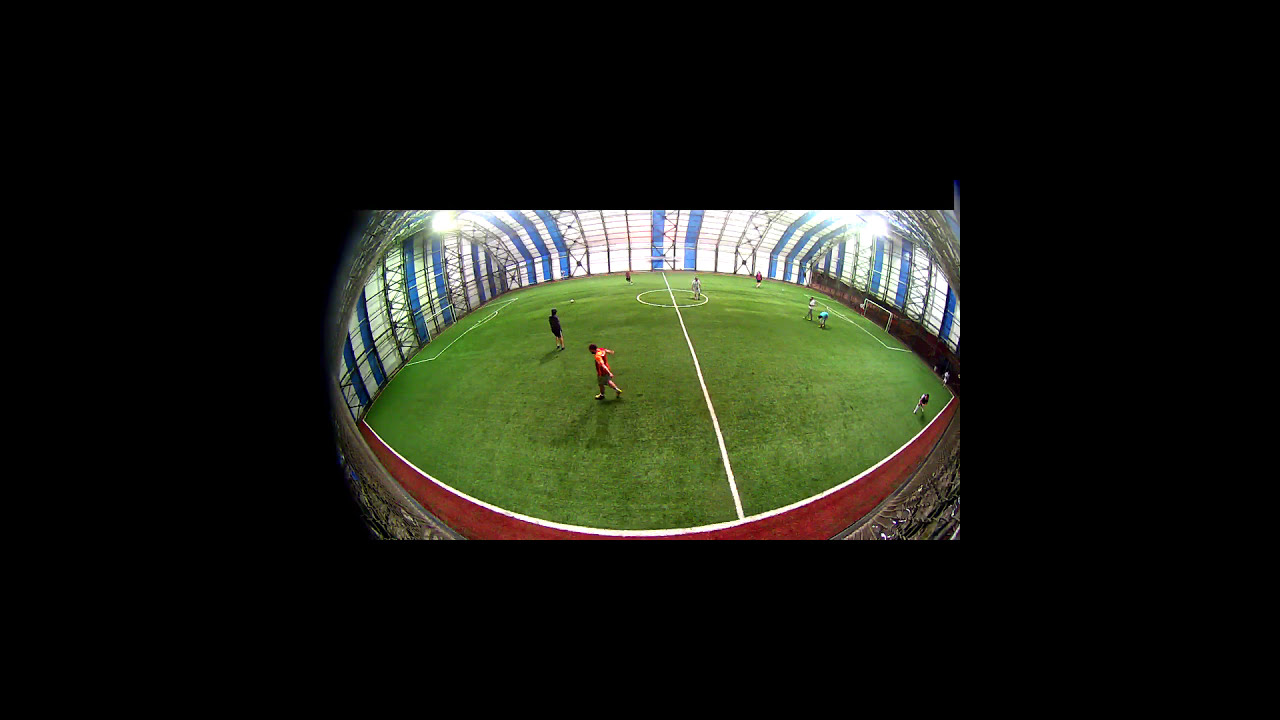The image depicts an indoor soccer field captured with a fisheye lens, giving it a distorted, circular appearance. The field itself is vividly green with clearly marked white lines and borders. Surrounding the field are the distinctive blue and white stripes of the building structure, which also features black outlines and lighting on either side. A reddish stripe, possibly a running track, encircles the field. Scattered across the field are about eight to ten players dressed in various colors—orange, black, blue, white, and light blue—suggesting a practice session rather than an actual game. Both soccer goals are visible, with one placed on either end of the field, and a soccer ball lies off to the left side. The players appear to be taking a break or involved in drills, contributing to the impression of an informal training session.